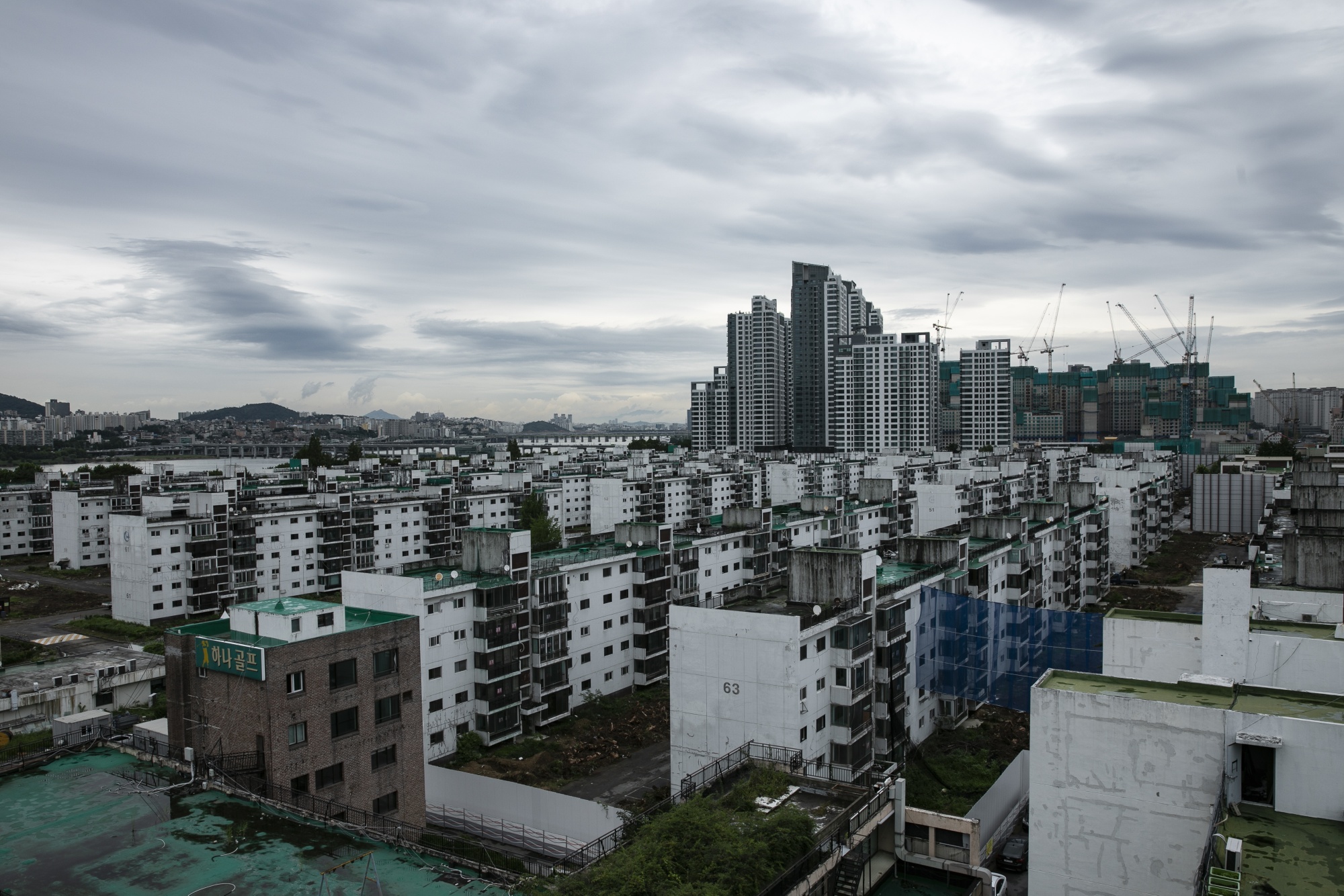This photograph captures a densely packed urban area filled with uniformly designed, white high-rise apartment buildings, characterized by their green painted roofs. The buildings appear dilapidated and weathered, with staining and a dingy appearance. Rows upon rows of these identical structures stretch across what seems to be an entire city block, each featuring small balconies. The bleak tone is emphasized by the overcast, cloudy sky, contributing to a sense of abandonment, as there are no people or vehicles present, and debris is visible on the ground, hinting at possible severe weather damage. In the left-hand side of the image, partially obscured writing in Korean reads "Hi-Ni-Gol." In the background, modern skyscrapers loom over the older buildings while cranes and construction equipment suggest ongoing repair efforts. Mountains and additional buildings are faintly visible in the distance, completing this somber urban landscape.